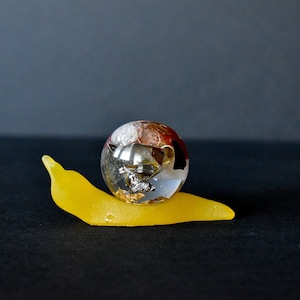This square photograph features a bright yellow, abstract form reminiscent of a banana or slug, made from a material that could be jello, clay, plastic, or even a dried fruit like mango. The yellow object, slightly leaning to its left, sits near the center of the image on a black or dark gray surface. The backdrop is a simple gray wall. Resting atop the yellow shape is a sphere, possibly a marble or glass ball, with chunks appearing chipped from its surface. This sphere has a mix of colors, including shades of brown, bluey-white, and glassy tones that create a distorted, almost room-like reflection within. The details of the sphere’s internal design are complex and hard to decipher. The entire composition is neatly contained within the small, square frame.